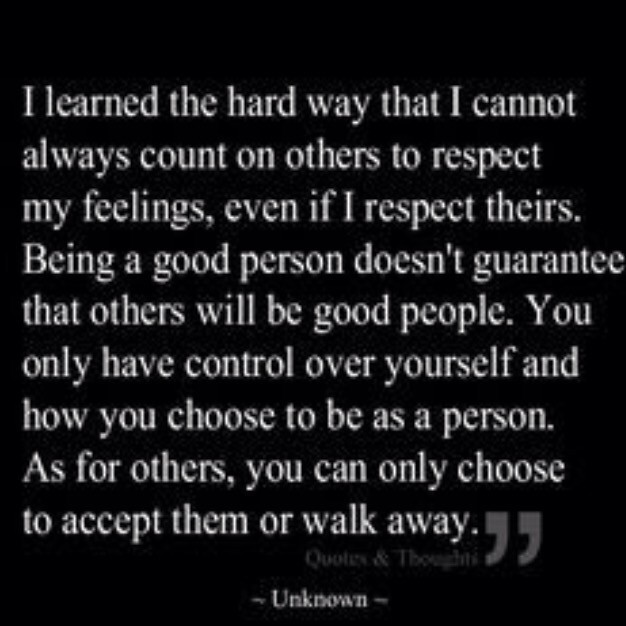The image depicts a graphic with a predominantly black background and a square format. The foreground features slightly pixelated, blurry white text that occupies most of the space. The text reads: "I learned the hard way that I cannot always count on others to respect my feelings, even if I respect theirs. Being a good person doesn't guarantee that others will be good people. You only have control over yourself and how you choose to be as a person. As for others, you can only choose to accept them or walk away." Below this poignant quote, in very pale gray text, the phrase "quotes and thoughts" is displayed. Flanking this phrase are two large quotation marks that are as tall as the words "away" and "thoughts" in the quote above. At the bottom center of the image, in white print, the source is credited as "unknown." The background appears mostly plain, but there might be subtle spirals or stripes, which could be optical illusions created by the text's fuzziness.